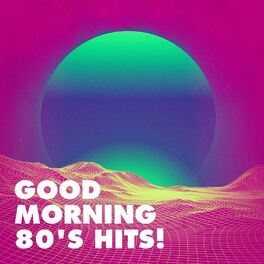This vibrant image appears to be a colorful flyer or poster for a radio station, featuring bold and vivid colors that evoke a nostalgic 80s aesthetic. The background of the image is dominated by a magenta square with a stylized, hilly terrain at the bottom that has a pink and red checkerboard pattern. Over this terrain, there is a striking yellow paint effect spilling over the edges, resembling sunlight illuminating the landscape.

In the center of the composition is a large, eye-catching circle that has a mint green color on its top and bottom portions, with a darker navy or possibly deep purple hue in the middle, creating the appearance of a planetary body. This planet-like circle floats above the terrain, enhancing the otherworldly feel of the image.

In the bottom left corner of the poster, bold white text reads "Good Morning 80s Hits!" This text stands out prominently against the backdrop, indicating it might be a tagline or slogan for a vibrant 80s hits radio station. The combination of bold colors and playful design elements exudes energy and nostalgia, making for an eye-catching and memorable visual statement.